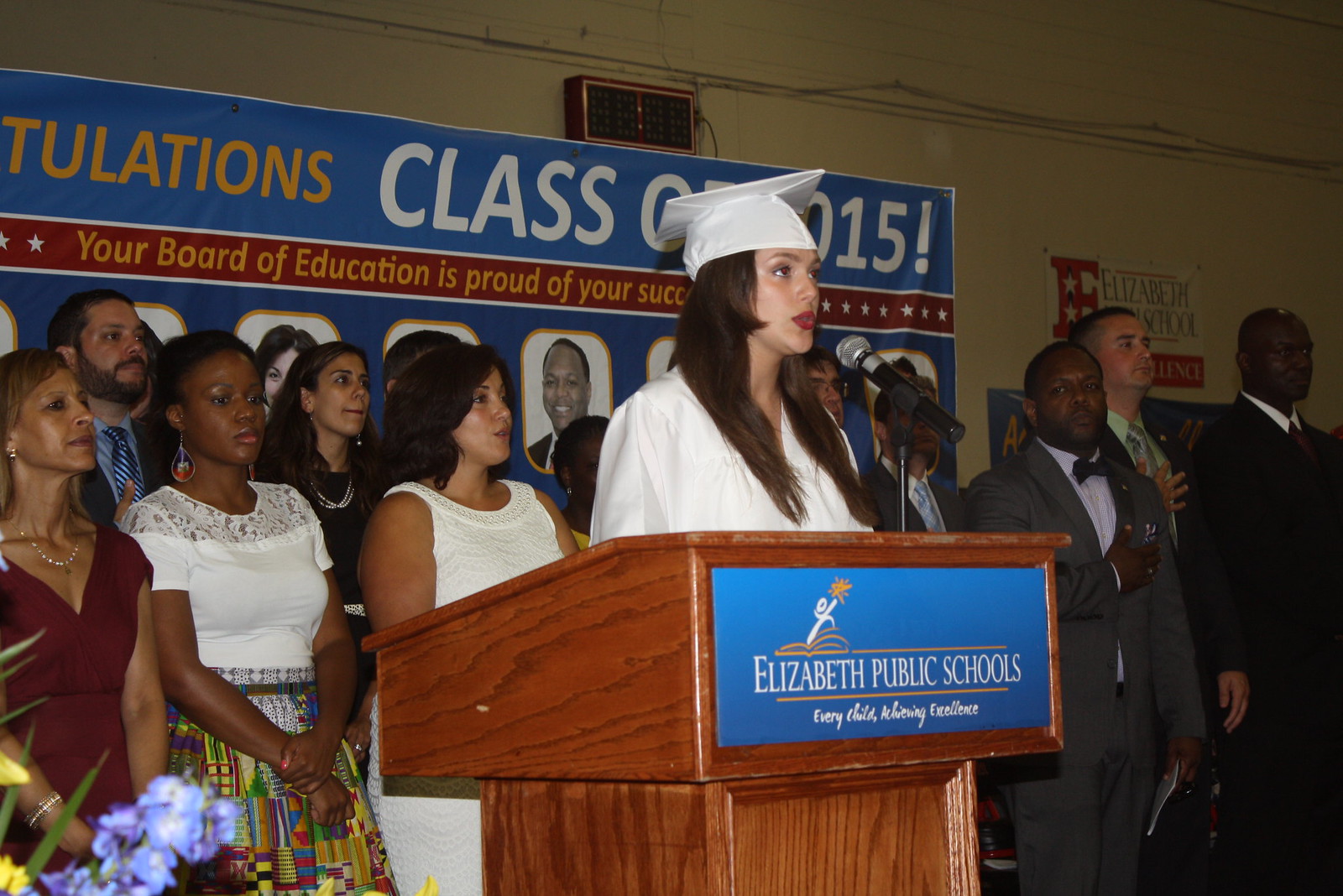The image captures a close-up view of a graduation ceremony at Elizabeth Public Schools. At the center, a young woman with long brown hair stands at a dark brown wooden podium, dressed in a white graduation gown and matching cap. She appears to be speaking into a black microphone held by a stand. The podium features a blue placard with white text that reads, "Elizabeth Public Schools. Every child achieves excellence."

Behind her, multiple people, possibly teachers or administrators, are standing and looking towards the right. The background is adorned with a large banner that says “Congratulations Class of 2015” in yellow text, slightly cut off at the edges. Below this, a red rectangular strip contains yellow text, partially obscured by the woman, which reads, "Your Board of Education is proud of your success." The image captures the celebratory atmosphere of the graduation with its detailed setting and elements.